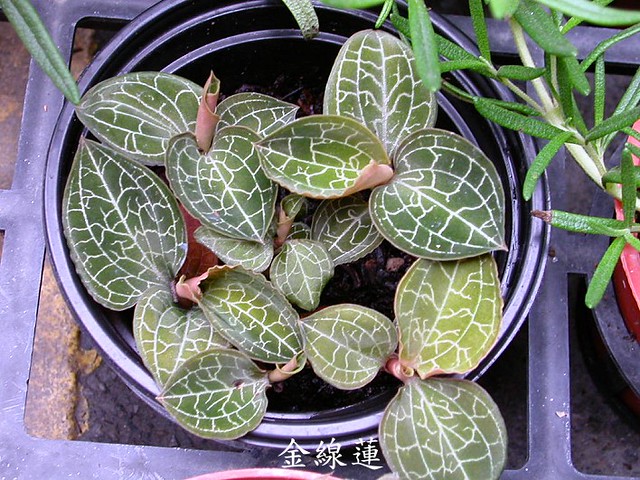The photograph depicts a potted plant with smooth, rounded, and large green leaves, each featuring irregular cream-colored lines forming a distinctive reticulate pattern. The plant is housed in a circular black pot filled with dark soil, and is placed outdoors in daylight, possibly on a black railing. On the right edge of the image, a glimpse of another potted plant with dark green leaves can be seen. At the bottom of the image, there are three Japanese characters written in white, overlaid in the center. The leaves of the main plant also have a slight curvature, indicating varying ages.